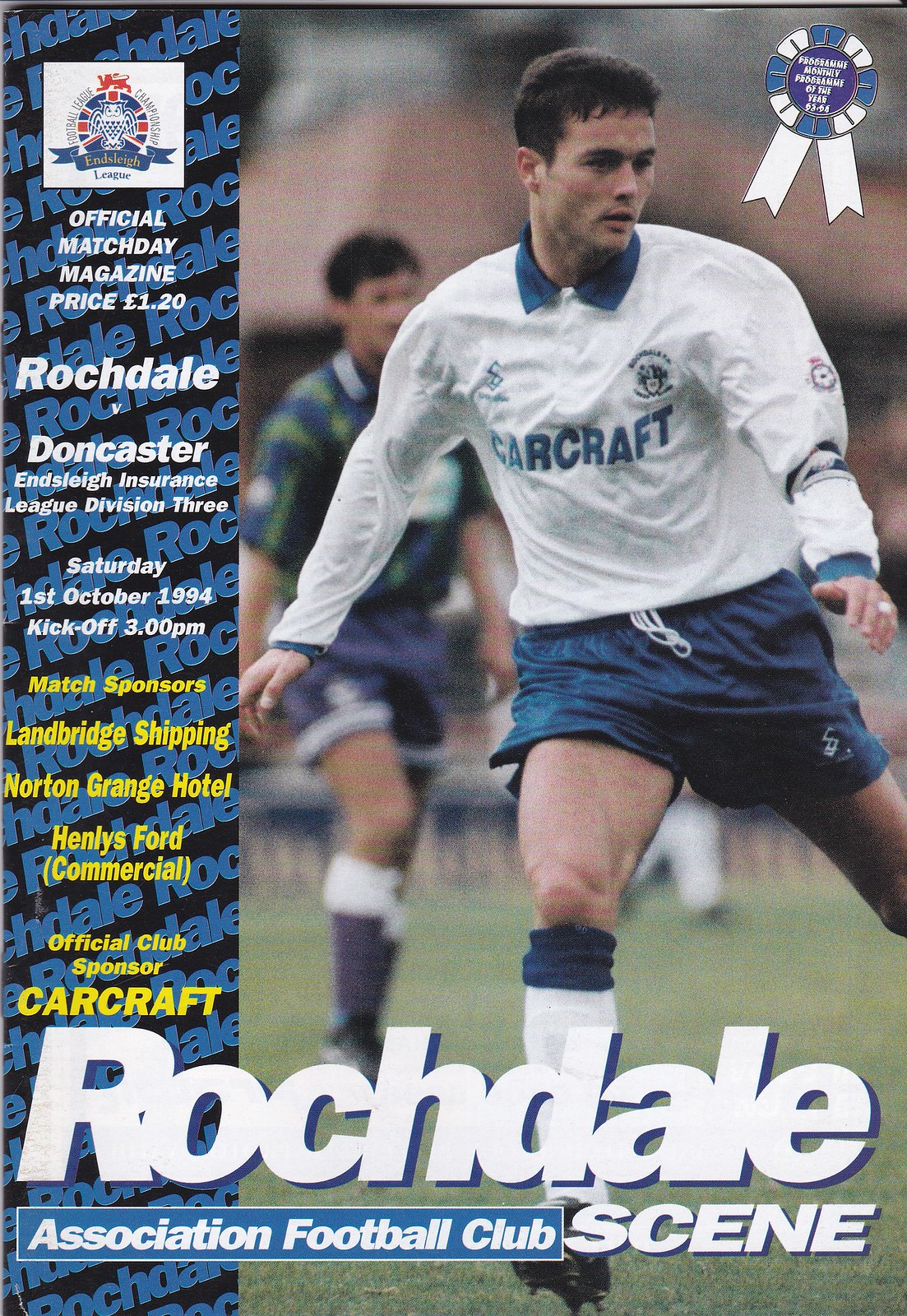This is an image of the official match day magazine for the Rochdale Association Football Club, titled "Rochdale Scene." The magazine features a dynamic cover with two soccer players prominently displayed. The player in the foreground, wearing a long-sleeved white jersey with "Carcraft" printed on the front, is dressed in blue shorts and white shin guards with blue trim. He's captured mid-action, seemingly moving towards the camera with his head turned slightly. Just behind him, another player is dressed in a blue and green striped jersey and dark blue shorts, sporting blue shin guards.

The top right of the cover displays a blue and white ribbon, while the left side features "Rochdale" repeatedly in blue text against a black background. Above this area is a logo in a white box with a crest. The bottom of the image reads "Rochdale Scene, Association Football Club" at the bottom in white text, set against a blue background. Additional details include the price of the magazine, £1.20 EUR, and the match information: "Official Match Day Magazine, Rochdale vs. Doncaster, Ensley Insurance League Division III, Saturday 1st October 1994, Kickoff at 3 p.m." The match sponsors listed in yellow are "Landbridge Shipping, Norton Grange Hotel, Henley's Ford Commercial," with Carcraft noted as the official club sponsor. The design also incorporates colors of white, blue, yellow, and green grass hues throughout.